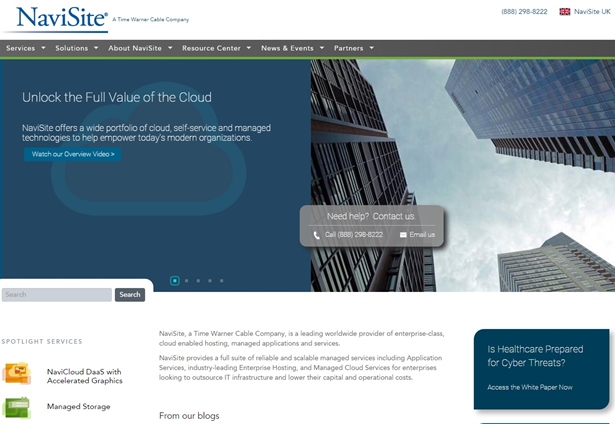A high-resolution screenshot of a professional healthcare technology website showcases its modern design and user-centric interface. On the right side of the image, an impressive photograph of skyscrapers captures attention, symbolizing growth and innovation. The central headline reads, "Unlock the Full Value of the Cloud," underlining the website's focus on advanced cloud solutions. NaviSite is highlighted as offering a broad portfolio of cloud self-service and managed technologies designed to empower today's modern organizations. At the bottom right corner, a thought-provoking tag prompts, "Is healthcare prepared for cyber threats? Access the white paper now," urging users to delve deeper into current industry challenges. The overall aesthetic of the website is meticulously crafted with high-quality visuals and a sophisticated color palette, reflecting a significant investment of time and effort to align it with contemporary industry standards. The eye-catching colors and polished design elements effectively draw the viewer's attention to essential details, emphasizing the website's dedication to excellence and innovation in healthcare technology.